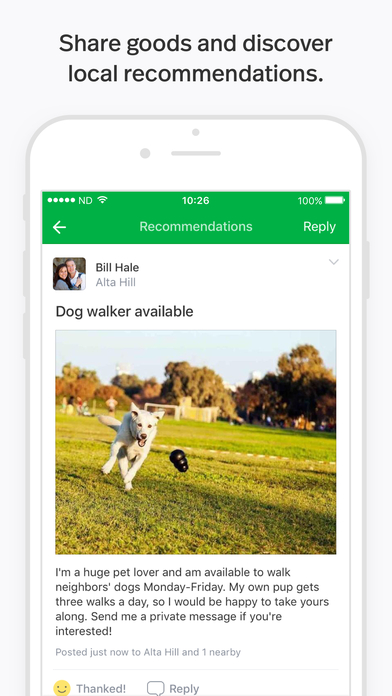A screenshot from a local community app, such as Facebook Neighborhoods or Nextdoor, features a clean white backdrop with promotional text at the top saying, "Share goods and discover local recommendations." Below this text, there is an image of a white smartphone displaying the app interface, with a green navigation bar at the top indicating the sections "Recommendations" and "Reply." The interface shows a recent post from a user named Bill Hill, located in Alta Hill, advertising dog-walking services.

In Bill Hill's post, there is a profile picture of a middle-aged man and woman, approximately 50 years old. Accompanying the post is a large, vibrant photo of a white dog energetically running on a grassy field, chasing a black ball, with a scenic background of lush green trees and a clear blue sky.

The post's caption reads: "I'm a huge pet lover and I'm available to walk neighbors' dogs Monday through Friday. My own pup gets three walks a day, so I'll be happy to take yours along. Send me a private message if you're interested." 

The post has just been uploaded to the Alta Hill section and another nearby neighborhood. It has received two engagement markers: one for "Thanks" and one for "Reply." This encapsulates an enthusiastic community member offering dog-walking services and seeking interested individuals.